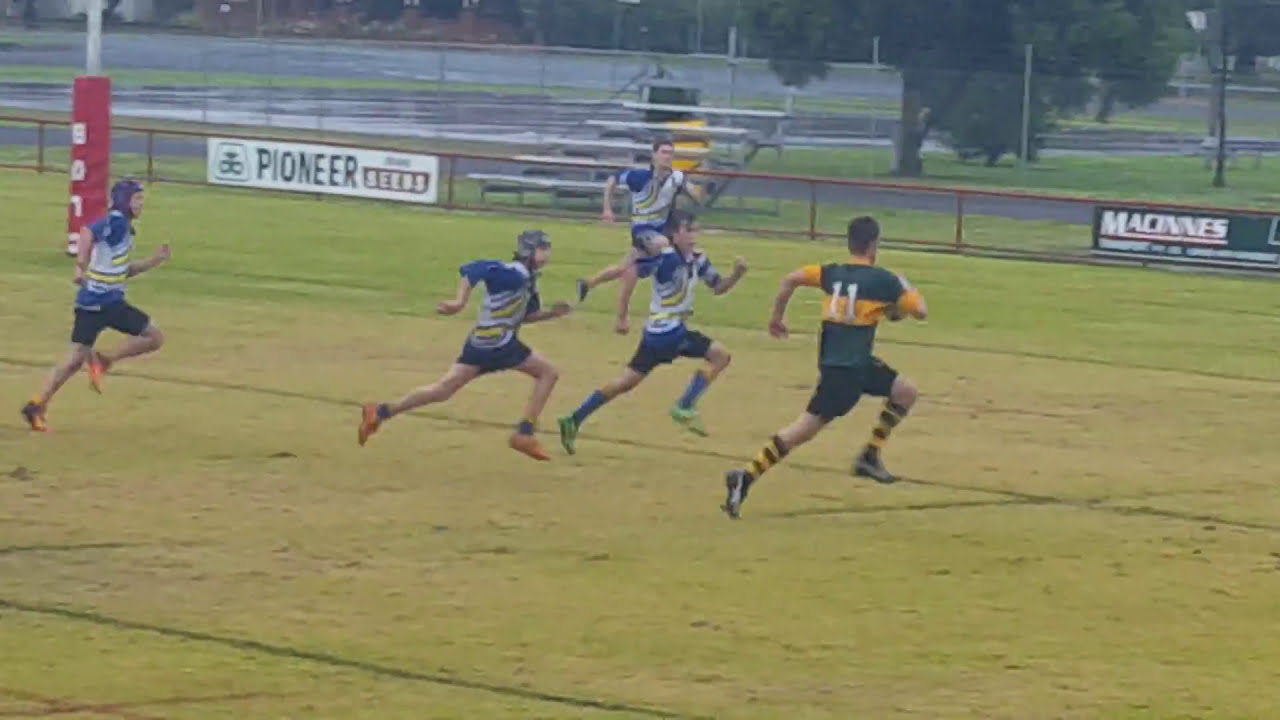The image captures a dynamic rugby match on a grassy field. At the center-right, a player wearing a green and orange striped jersey with the number 11 on the back is seen running away from the camera while clutching the ball. He dons black shorts, yellow and black striped socks, and black shoes with a white stripe. Chasing him from the left are four opponents dressed in blue-sleeved jerseys with white centers and yellow and black stripes, paired with black shorts. The field features thin black lines running horizontally and is surrounded by various elements: to the left, a pole with a protective cushion, and in the background, a short gray fence adorned with a Pioneer Seeds banner on the left and another sign reading 'Macines' on the right. Beyond the fence, there's a gray bleacher, a wet parking lot, another fence, and a solitary tree against a backdrop of dense green vegetation.